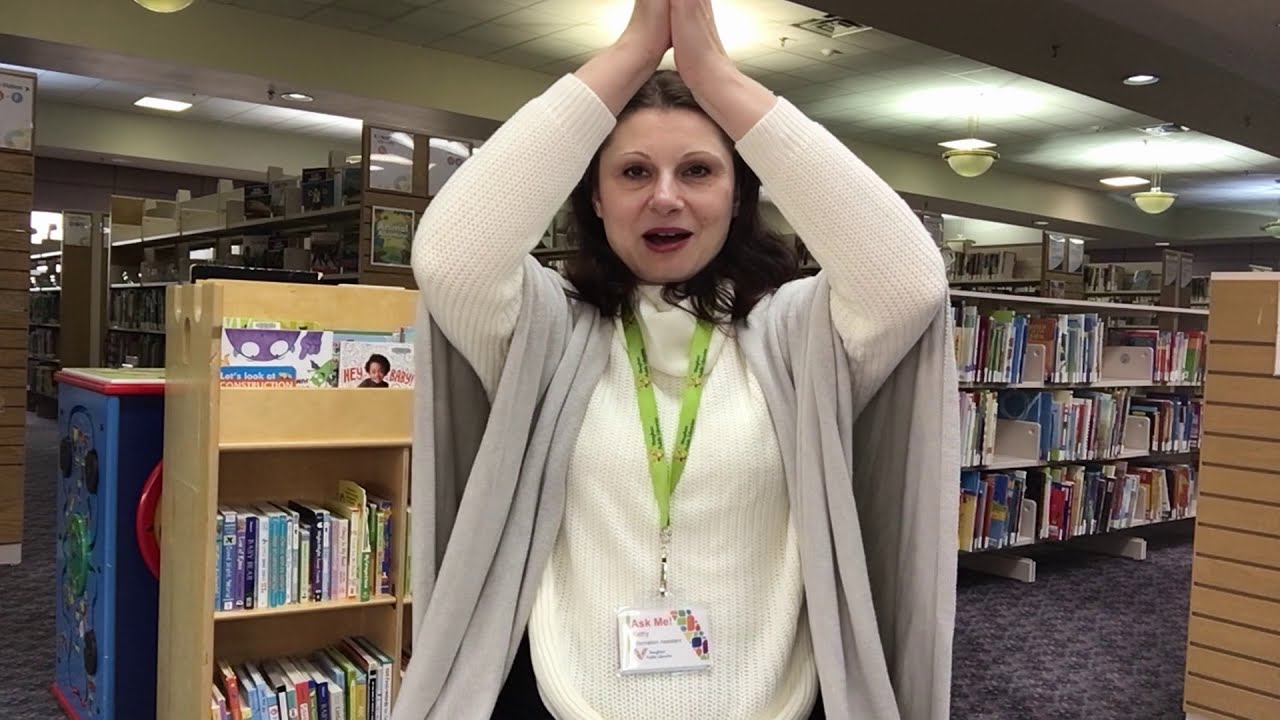In the center of the frame stands an older Caucasian woman, likely in her 40s or 50s, inside a dated library with multicolored patterned carpet. She has short, shoulder-length brown hair and is dressed in a long-sleeve cream-colored sweater with a gray shawl draped over her shoulders. The woman wears a green lanyard bearing a badge that reads "Ask Me," indicating that she is probably a librarian or volunteer. Her arms are raised above her head, palms pressed together in a gesture resembling a shark fin or praying motion, and her mouth is slightly open, as if she is speaking. Behind her, there are various shelves filled with children's books and, in the distance, larger library stacks. Additionally, there’s a wooden rolling cart with several rows of books on the left side of the image. Overhead, the ceiling lights and other library fixtures can be seen.